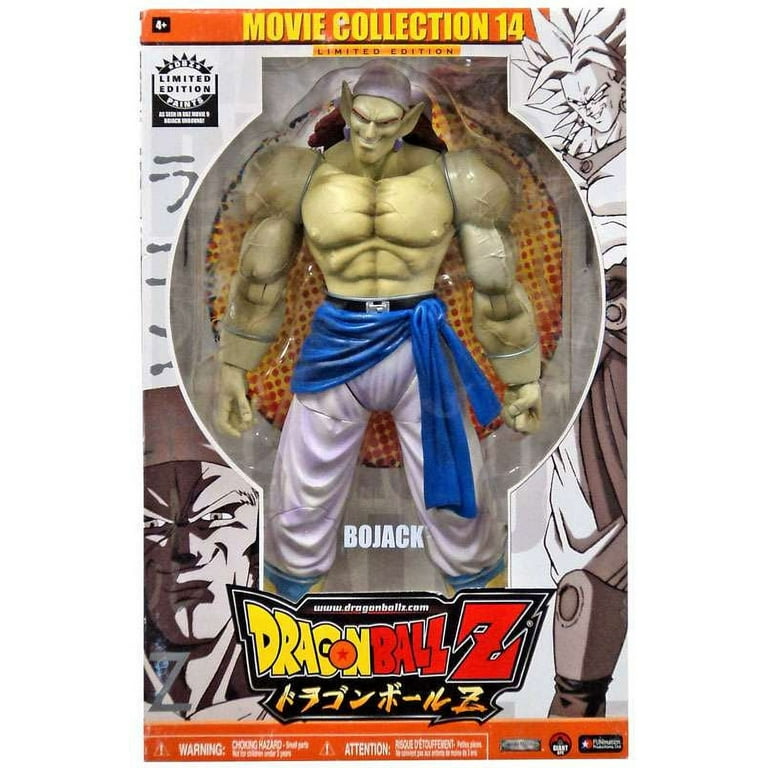In this detailed full-color vertical marketing image, the central focus is on a limited edition action figure from the Japanese anime Dragon Ball Z, specifically featuring the character Bojack. The top of the packaging prominently displays a red banner with yellow text reading "Movie Collection 14" and “Limited Edition” in black text beneath it. Bojack, the green-skinned, muscular creature with elf-like ears, is encased in a clear plastic display. He wears white pants and has a blue sash tied around his waist, secured with a black belt and a silver clasp. The figure also sports a light purple cap on his head. His well-defined muscles are accentuated by vein ridge lines, and his stance is commanding with arms pointed down. Flanking the figure are black and white illustrations of other Dragon Ball Z characters, adding to the dynamic presentation of the packaging. At the bottom center of the packaging, "Dragon Ball Z" is visibly printed in bold letters, with "Dragon" in yellow and "Ball Z" in red.